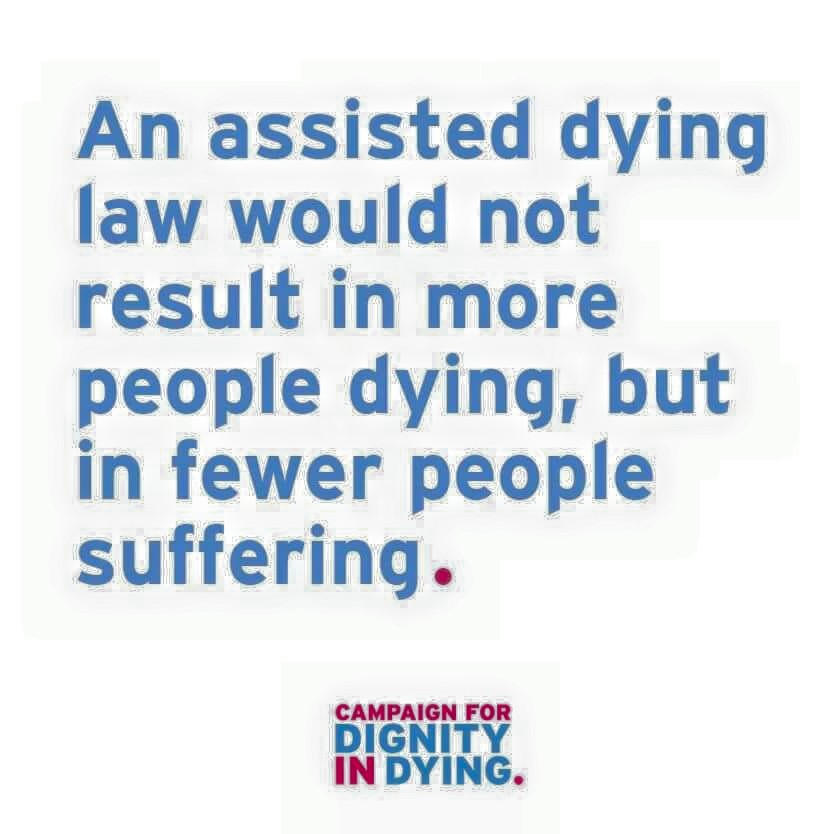The image depicts a white background with a prominent blue text message that reads: "An assisted dying law would not result in more people dying, but in fewer people suffering." The sentence ends with a distinctive red period. Below this message, in a smaller rectangle, there is a set of words that appear to indicate the sponsoring organization. This text reads "Campaign for Dignity in Dying," where "Campaign for" and "in" are in red, while "Dignity" and "Dying" are in blue, all capped with a final red period. The combined messages emphasize support for an assisted dying law, advocating that it would reduce suffering rather than increase mortality.